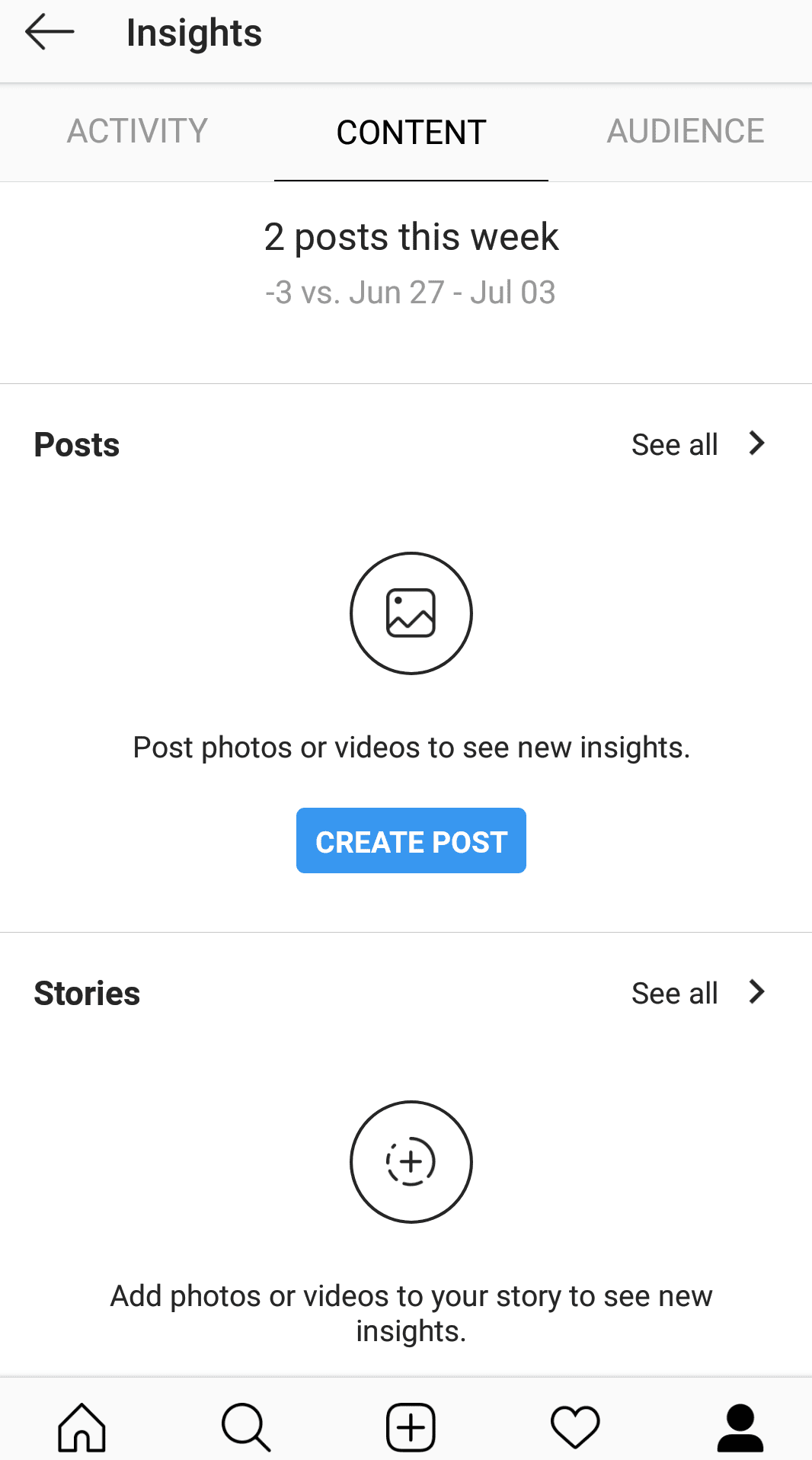This is a detailed caption for the image:

---

A vertical, smartphone-style screenshot with a predominantly white background, likely from a social media analytics or insights page. At the top of the screenshot, two long grey rectangular bars are separated by a slightly darker grey line. An arrow icon pointing to the left and the word "Insights" in black text is visible beside these bars.

Below this header, three categories labeled “Activity,” “Content” (which is bolded and underlined), and "Audience" are displayed. In the main section of the image, a line of black text reads: "2 posts this week, -3 compared to June 27 to July 3," with a thin line separating this section from the next.

On the left side, the word "Posts" is in bold black, while "See All" is written in less bold text to the right, accompanied by an arrow pointing to the right. Below this, centered, is a circle containing a photo icon and the text "Post photos or videos to see new insights." A blue button with white text labeled "Create Post" is beneath this section, separated by another thin line.

Further down, the word "Stories" is in bold black text. An option to "See All" is available with a middle-aligned circle featuring a plus sign and the message "Add photos or videos to see your story insights."

At the bottom of the screenshot are familiar icons for home, search, post creation (plus sign), notifications (heart symbol), and user profile (person icon).

---

This caption provides a detailed and organized description of the image elements and their layout, suitable for a reader seeking a clear understanding of the visual content.